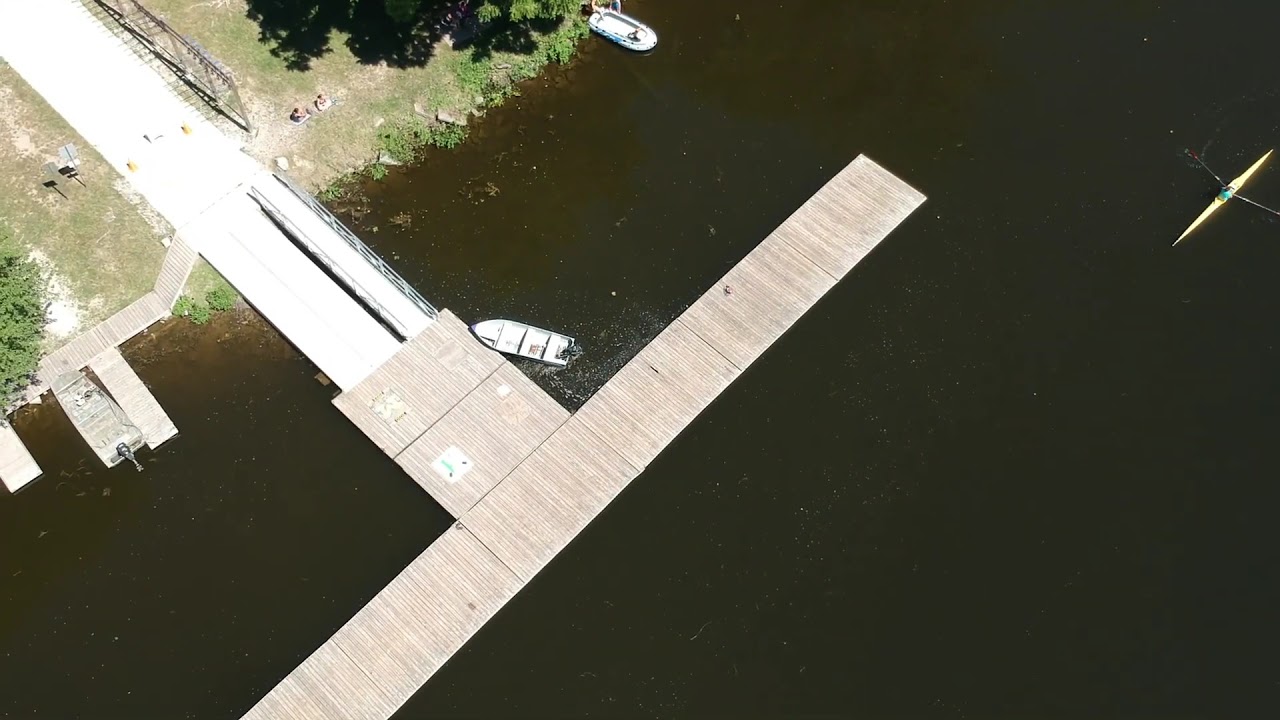This overhead image captures a wooden dock extending diagonally from the bottom left to the upper right, perched over a murky green body of water. The dock features a central square segment leading to a white-colored walkway with considerable reflections, which further branches out into a wheelchair ramp with safety barriers. In the upper right corner, a yellow boat can be seen with an individual rower in a teal shirt using oars. To the left, touching the dock at the front, there's a white boat with a black engine. Further towards the upper center-left, another white inflatable raft is visible. On the land in the upper left corner, the ground is a mix of grass and dirt, surrounded by spotty vegetation, bushes, and some trees casting shadows. The scene appears to be a serene lakeside area with no discernible text, emphasizing the natural and constructed elements harmoniously blending together.